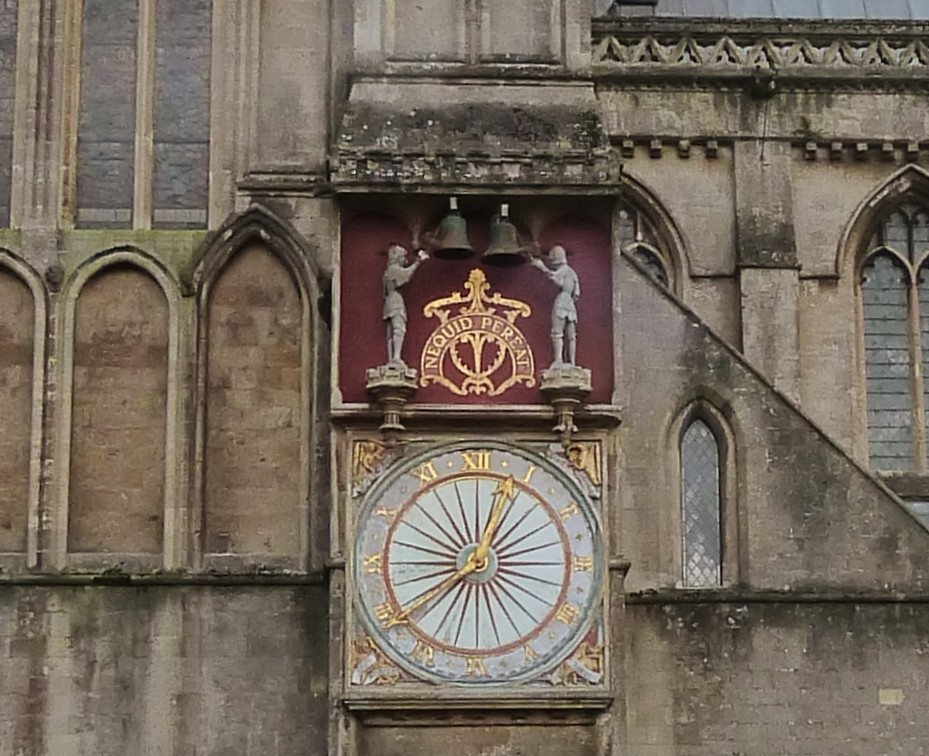This photograph depicts an intricately designed clock tower integrated into an ancient, ornate church, likely situated somewhere in Europe. The centerpiece is a large clock with gold Roman numerals showing the time as 12:40. The clock is mounted on an ornamental square base adorned with a simple sunburst design at its center.

Above the clock, there is a decorative cupola featuring a small concrete pergola. This area also houses two large bells, each flanked by statues of men who seem poised to ring them. The backdrop behind the bells and statues is a burgundy panel, embellished with a gold crest bearing the inscription "Nequid Perat."

The architectural style of the building is striking, with its tall, thin, pointed windows, some of which showcase intricate stained glass while others are bricked in, likely indicating various stages of renovation throughout the ages. The stone used in the church's construction appears to be quite old, adding to the historic charm of the structure. The overall design is highly ornate, emanating a sense of reverence and timelessness, characteristic of historic European churches.